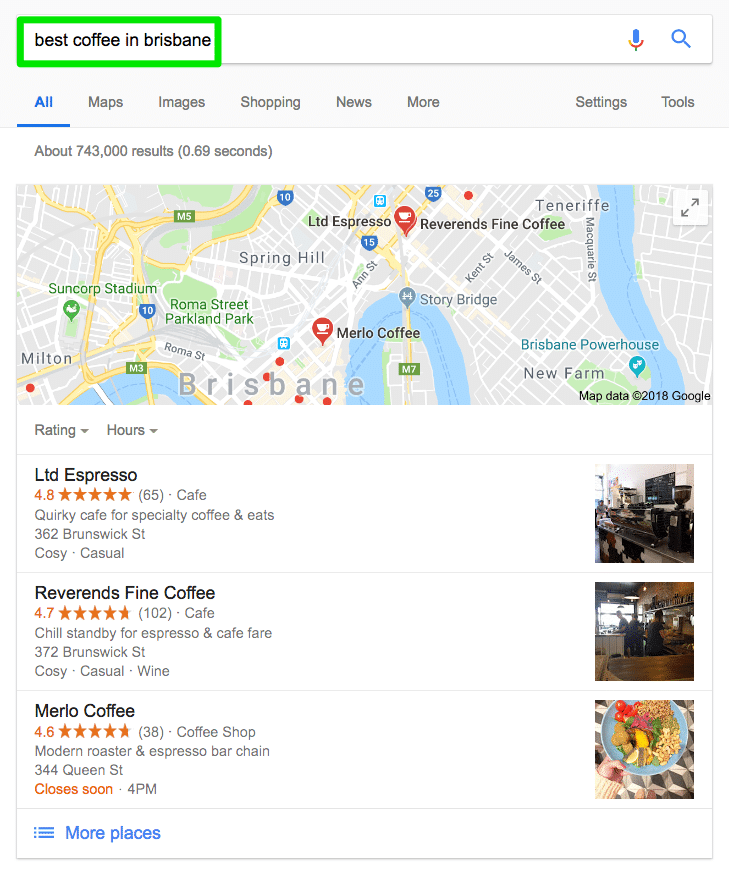The vertical image captures a search result page from a website, likely accessed on a computer or smart device, displaying the query "best coffee in Brisbane." The top part of the page features a light gray strip containing a white search bar with the query text highlighted by a thick green rectangular box. Within the search bar, both the microphone icon and the magnifying glass icon are visible.

Beneath the search bar, an array of options is presented in blue, all highlighted and underlined, including "All," "Maps," "Images," "Shopping," "News," "More," "Settings," and "Tools."

The search yields approximately 743,000 results, achieved in a swift 0.69 seconds. Below this introductory information is a map pinpointing recommended coffee spots in Brisbane, each location annotated with ratings and operational hours, allowing users to filter results accordingly.

Highlighted cafes include:
- **Limited Espresso**, boasting a 4.8-star rating from 65 reviews, accompanied by a brief description, address, and a note on its ambiance (cozy, casual, or formal).
- **Reverends Fine Coffee**, holding a 4.7-star rating based on 102 reviews.
- **Merlo Coffee**, rated 4.6 stars from 38 reviews.

At the bottom is a clickable blue link labeled "More places," inviting users to explore additional options. Each listed coffee shop comes with an image on the far right, providing a visual representation of the respective establishments.